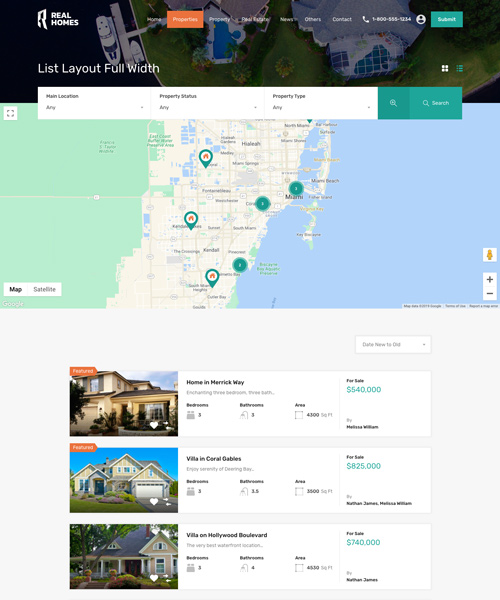A high-angle view captures an exquisite waterfront property available for real estate. The property features a spacious house with an inviting swimming pool and is situated on a scenic point surrounded by lush green lawns. Adjacent to the property, a dock accommodates a large boat and a smaller vessel, enhancing the luxurious appeal.

The image appears to be part of a real estate template with the header "Real Homes" and a stylized "R" logo. A navigation menu at the top includes options such as Home, Properties, Property, Real Estate, News, Others, Contact, along with a phone number and a profile icon. The 'Properties' tab is highlighted in orange.

This first layout showcases a full-width mock-up with search options accompanying the main location, property status, and property type filters. A green-teal button labeled "Search" is positioned to the right. Below this section, a visual representation of a Google Map is inlaid and stylized, offering Map and Satellite viewing options. The search results section displays selections in a color scheme of greenish-teal and orange.

Featured properties are listed beneath this, including "Home and Merrick Way,” “Villa and Coral Gables," and "Villa and Hollywood Boulevard." Each listing includes detailed information about the number of bedrooms, bathrooms, square meters, and price. The top two listings are marked with orange "Featured" banners and the prices in teal: $540,000, $825,000, and $740,000 respectively, alongside a "For Sale" status.

This sophisticated template effectively showcases the breathtaking properties, catering to prospective buyers with comprehensive details and an elegant design.